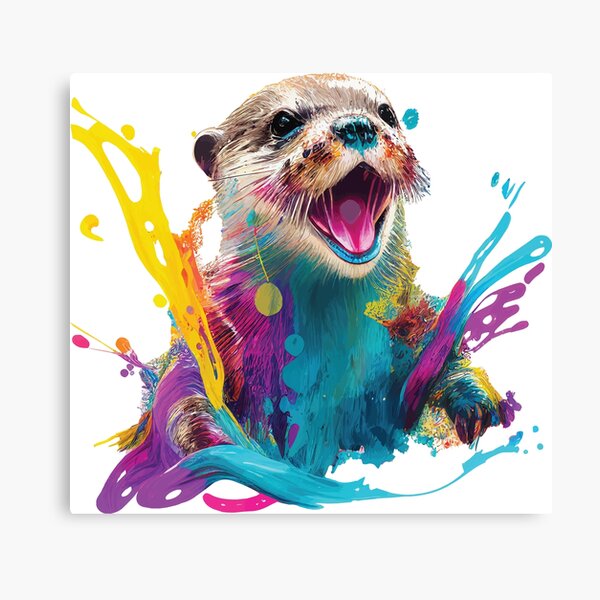An expressive painting on a white canvas features a vibrant portrait of a river otter, characterized by its light brown fur and distinct facial markings. The otter's face is animated with an open mouth revealing a pink tongue, small dark eyes, a small nose, and small ears, capturing a sense of joyful exuberance. Colorful splashes of blue, teal, purple, yellow, red, and orange cascade down its shoulders and chest, blending into one another in a dynamic and playful manner reminiscent of pop art. These splashes create a striking visual effect, as if someone poured a bucket of colors over the otter, with the paint flowing around its body and onto the white background. Beneath the otter, a long blue wavy stripe interwoven with purple, pink, and a bit of green, completes the composition, enhancing the sense of motion and liveliness in this vividly imaginative artwork.